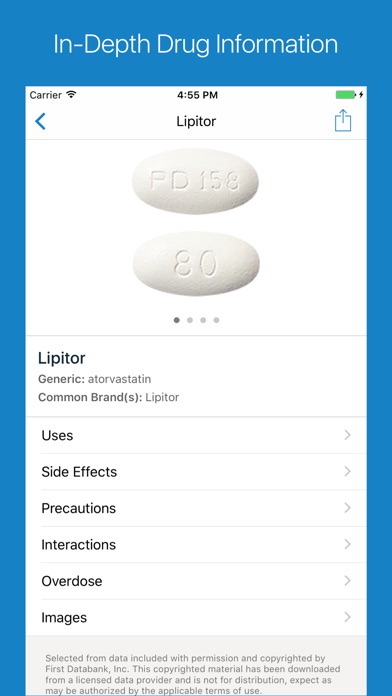The image features a predominantly blue background encompassing the top, left, and right sides. In the center, "In-Depth Drug Information" is prominently displayed. Below this header, there is a long white rectangular box. In the left portion of this box, the word "Carrier" is visible, while in the middle, the time reads "4:56 PM." To the right, a green bar indicates a full battery.

Beneath the time, the text "Lipitor" appears, referring to the medication in focus. The image showcases two pills: the first one, etched with "PD 158," is displayed at the top, and the second pill, etched with "80," is shown below it. Both pills are off-white in color.

Following the pill images, the caption "Lipitor (generic: atorvastatin)" is noted. Additionally, "Lipitor" is identified as a common brand name, highlighted with the letter "s" in parentheses next to it.

Continuing downwards, there are various categories listed: "Uses," "Side Effects," "Precautions," "Interactions," "Overdose," and "Images." These sections presumably offer detailed information about the medication. The description concludes with these categories, emphasizing the comprehensive nature of the drug information provided.